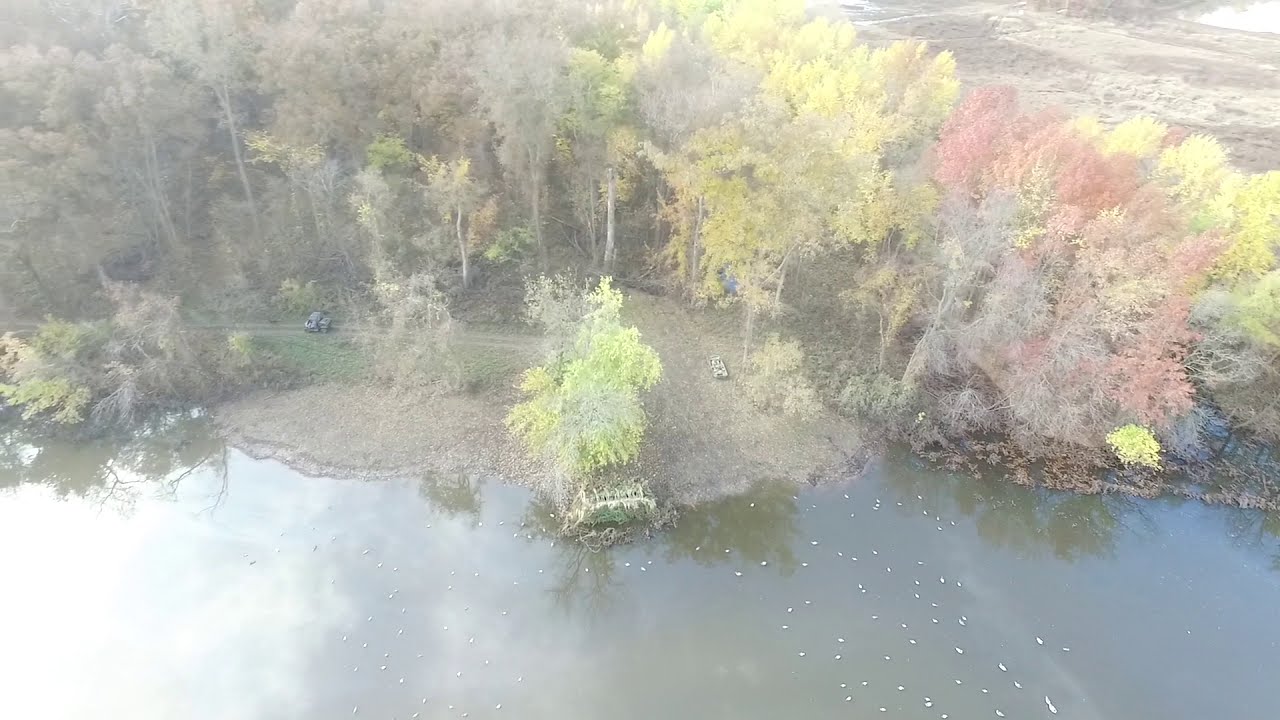The aerial image captures the edge of a lake bordered by a wooded area adorned with the colors of autumn. The water is a muddy brown, dotted with numerous white specks that suggest the presence of either birds or fish. Surrounding the lake, the landscape is dominated by trees with leaves in shades of yellow, red, and orange, interspersed with some barren, gray trees indicative of the season. Along the shoreline, a small vehicle is visible on a path, adding a touch of human activity to the natural setting. In the center-right of the image, a boat can be seen on the gravel near the water's edge. The top portion of the image reveals a dusty, dirty field stretching out from the dense woodland down to the waterline, with additional areas of water possibly part of a larger lake. The serene yet dynamic scene is alive with the signs of wildlife and subtle hints of human presence, highlighting the intricate interplay between nature and civilization.